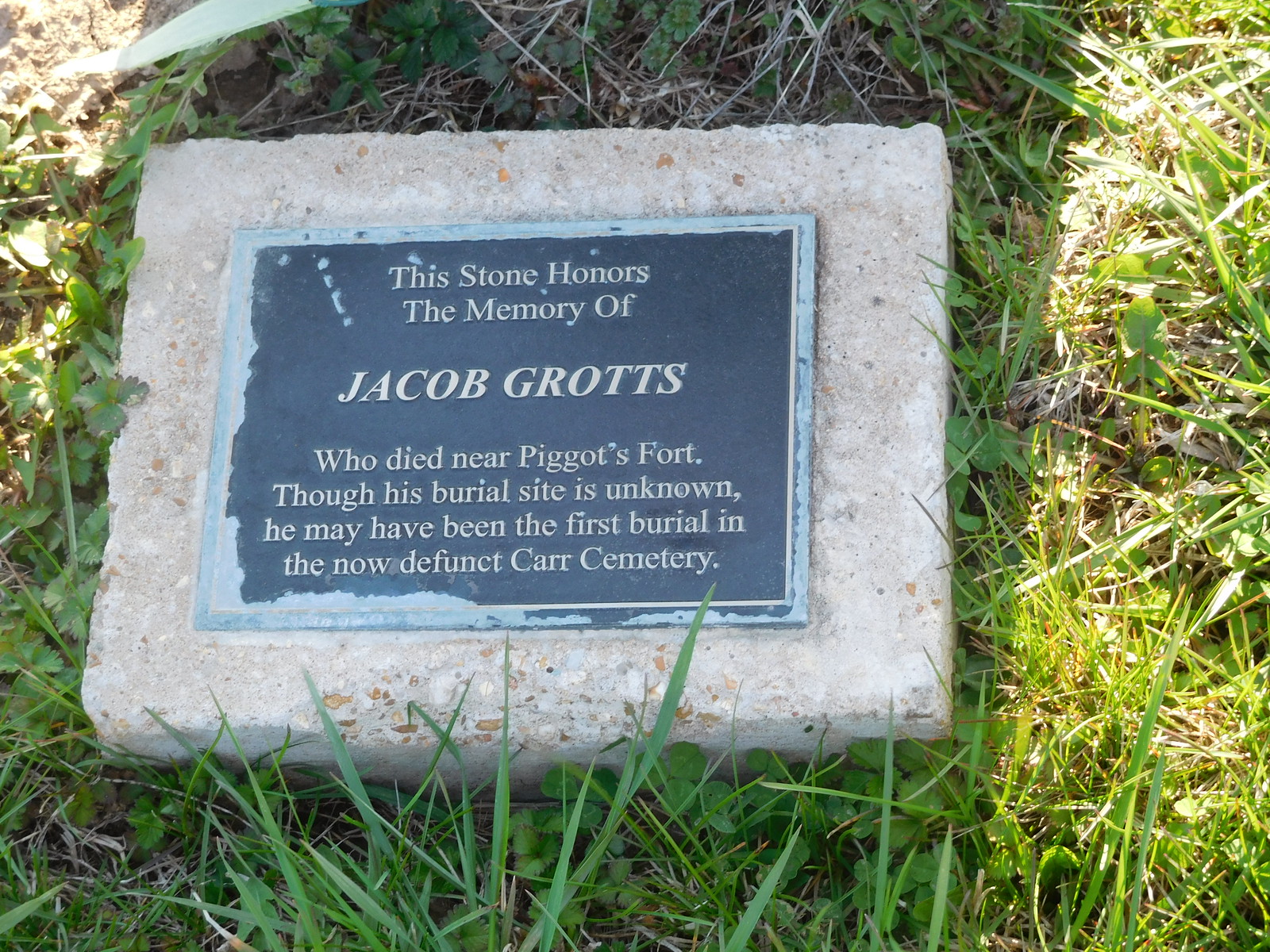The image is a tall, wide, rectangular photograph showcasing a memorial stone. The stone, resembling a headstone, lies slightly to the left of the center on a patch of green grass mixed with weeds and flowers. The stone itself is rectangular, wider than it is tall, and composed of light beige or gray granite. At the center of the stone is a wide, rectangular plaque made of dark brown, blackish metal with a greenish or bluish tinge around the borders. The inscription on the plaque is written in a gold or white font, which reads: "This stone honors the memory of Jacob Grotz, who died near Piggott's Fort. Though his burial site is unknown, he may have been the first burial in the now-defunct Carr Cemetery." The photograph also captures the shadow of the person taking it, which falls over the entire stone, adding depth to the scene.